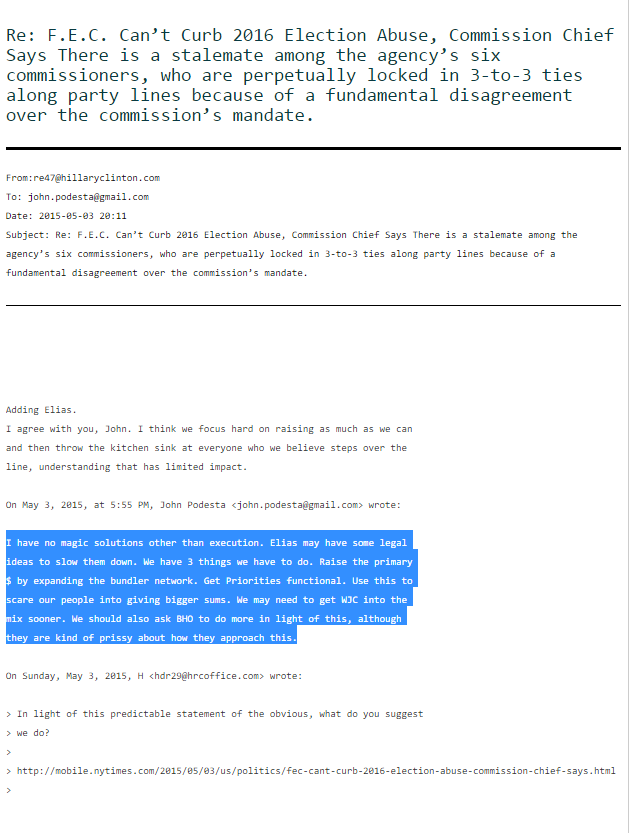This image appears to be a screenshot taken from someone's cell phone, capturing an email displayed on the screen. At the top of the image, there is a headline from an article titled "Election Abuse: Commission Chief Says There Is a Stalemate Among the Agency's Six Commissioners." The text describes a deadlock within the commission, with commissioners split into three-to-three ties along party lines due to fundamental disagreements on the commission's mandate.

Further down, the email excerpt shows correspondence involving Hillary Clinton's email address (hilaryclinton.com) and John Podesta (johnpodesta@gmail.com), dated May 3, 2015, at 8:11 PM. The email also mentions another recipient, Marc Elias, and contains a highlighted paragraph that seems to have been the primary focus. 

The highlighted portion of the email reads: "I have no magic solution other than execution. Elias may have some legal ideas to slow them down. We have three things we have to do: raise the primary money by expanding the bundler network, get priorities functional, and use this to scare our people into giving bigger sums. We may need to get WJC into the mix sooner. We should also ask BHO to do more in light of this, although they are kind of prissy about how they approach this."

This detailed screenshot provides an insight into the internal communications and strategic discussions among key political figures, highlighting the challenges and tactical considerations of campaign management.